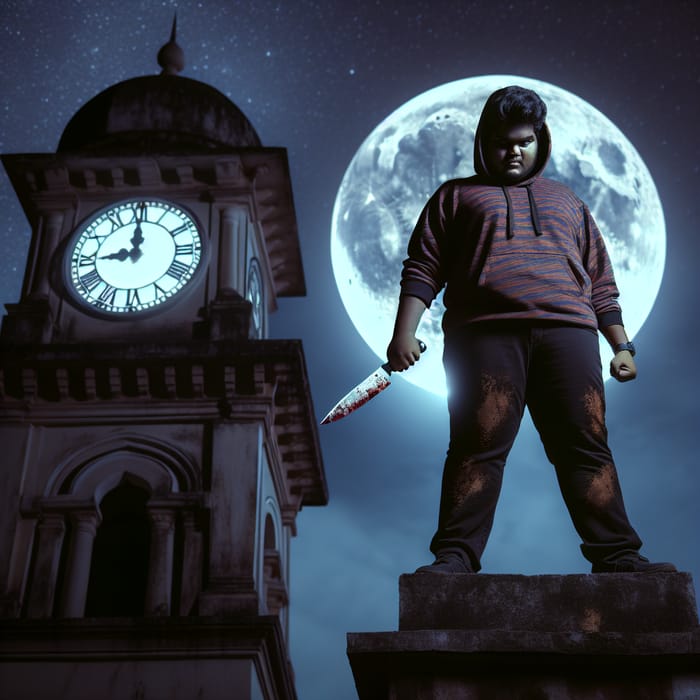The image depicts an AI-generated or drawn scene featuring a young man, possibly of Mexican or Indian descent, standing on a gray stone podium. He is wearing a burgundy hoodie with navy blue stripes, hood up over his wavy black hair, and black pants with brown mud stains or bleach marks. His right hand holds a blood-stained kitchen knife, and his left hand is clenched into a fist, adorned with a black watch. The man's expression is menacing, contributing to an overall ominous atmosphere.

Behind him, a large, full moon illuminates the dark blue, star-filled sky, which also contains a few visible clouds. To the left of the image stands a prominent stone clock tower with a domed roof, a white clock face with black Roman numerals, showing the time as nine o'clock. The clock tower features a glowing white face and an archway below it. The combination of the moonlit sky, the clock tower, and the young man with a bloody knife gives the scene a tense and eerie feeling.